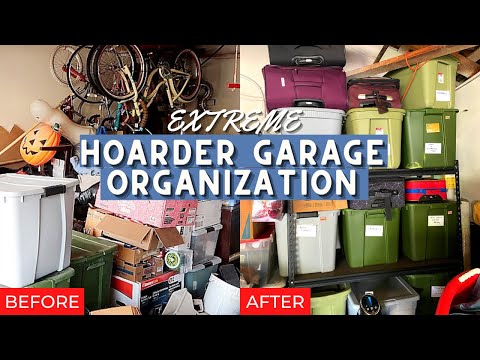The image features two photographs side-by-side, with a black bar at the top and bottom and text emphasizing a dramatic before-and-after transformation of a garage. The central text reads "EXTREME" in italicized white letters and "Hoarder Garage Organization" in bold white letters within a blue box. 

The left photograph, labeled "BEFORE" in a red-highlighted box with white text, shows a cluttered, chaotic garage. Bicycles hang from the ceiling, a plastic orange pumpkin with a black face is visible, and there are numerous cardboard and plastic boxes scattered and triple-stacked alongside other junk. Beige walls form the background.

The right photograph, marked "AFTER" in a similar red-highlighted box with white text, displays a well-organized garage. Neat metal shelving units hold labeled tote boxes, luggage bags, and other items arranged meticulously up to the ceiling. The transformation highlights extreme organizational efforts to clear the clutter and create a systematic, tidy space.